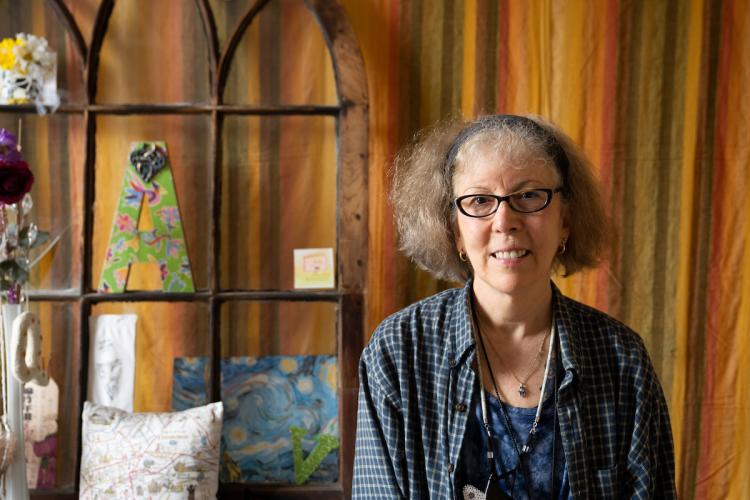The photograph features a middle-aged woman, likely in her 50s or 60s, positioned on the right-hand side of the frame. She has grayish-brown, slightly frizzy hair held back with a black headband and wears narrow, oval, black-framed eyeglasses. She is dressed in a blue patterned t-shirt underneath an open, checked button-down shirt. Around her neck, she has a small pendant on a chain and a stethoscope. The woman is smiling warmly, her mouth slightly open, as she looks directly at the camera.

In the background, the walls are adorned with striped patterns in shades of orange, green, yellow, and brown, which might be fabric hangings or wallpaper. On the left side of the photo, a shelving unit divided into three large arches is visible. Each arch contains three shelves filled with various objects. The top left shelf holds a flower arrangement, while the center holds a large decorated letter A and a light-colored pillow with gray decorations. The bottom shelf features another piece of artwork, including a small painting with a prominent letter V, surrounded by blue and white swirls and yellow dots, accompanied by an unreadable placard above it. The vibrant and warm ambiance suggests the setting is an art studio or a creatively decorated space.